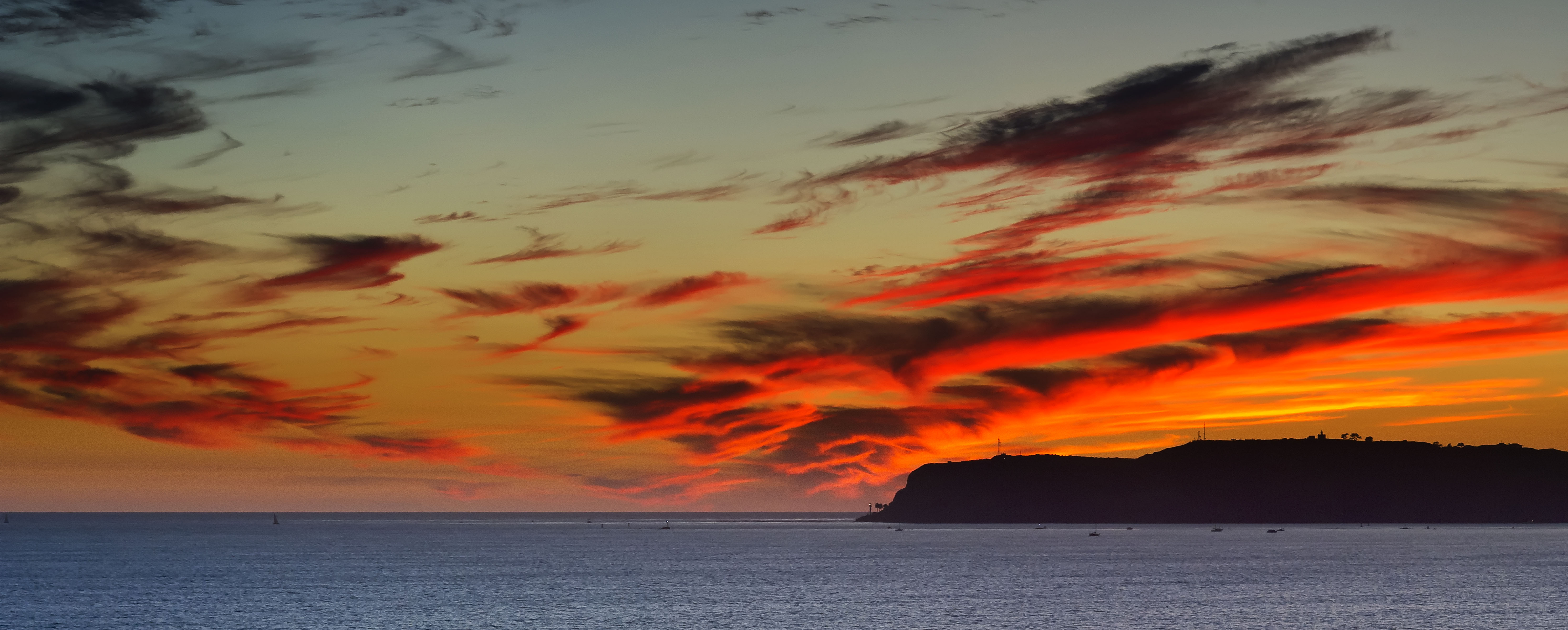This panoramic photograph captures a dramatic sunset over an expansive body of water, possibly an ocean or a great lake. The bottom portion of the image shows a clear, grayish-blue expanse of water. A silhouetted land feature protrudes from the right side, housing some trees and tall posts that may be part of a distant house, though all is indistinct due to the distance. Above this, the sky boasts a breathtaking array of colors: fiery oranges and blood reds dominate, creating an effect reminiscent of lava flowing through the sky. Wispy clouds scatter across the left side, while larger, more substantial clouds loom on the right, their dark forms tinged bright orange. The sky transitions from a grayish teal at the top to vivid orangish hues, capturing the essence of a splendid sunset. Boats float gently on the water, emphasizing the serene yet vibrant scene. This image is a stunning representation of nature's grandeur, drawing the eye to the magnificent, colorful sky while providing a tranquil view of the water below.